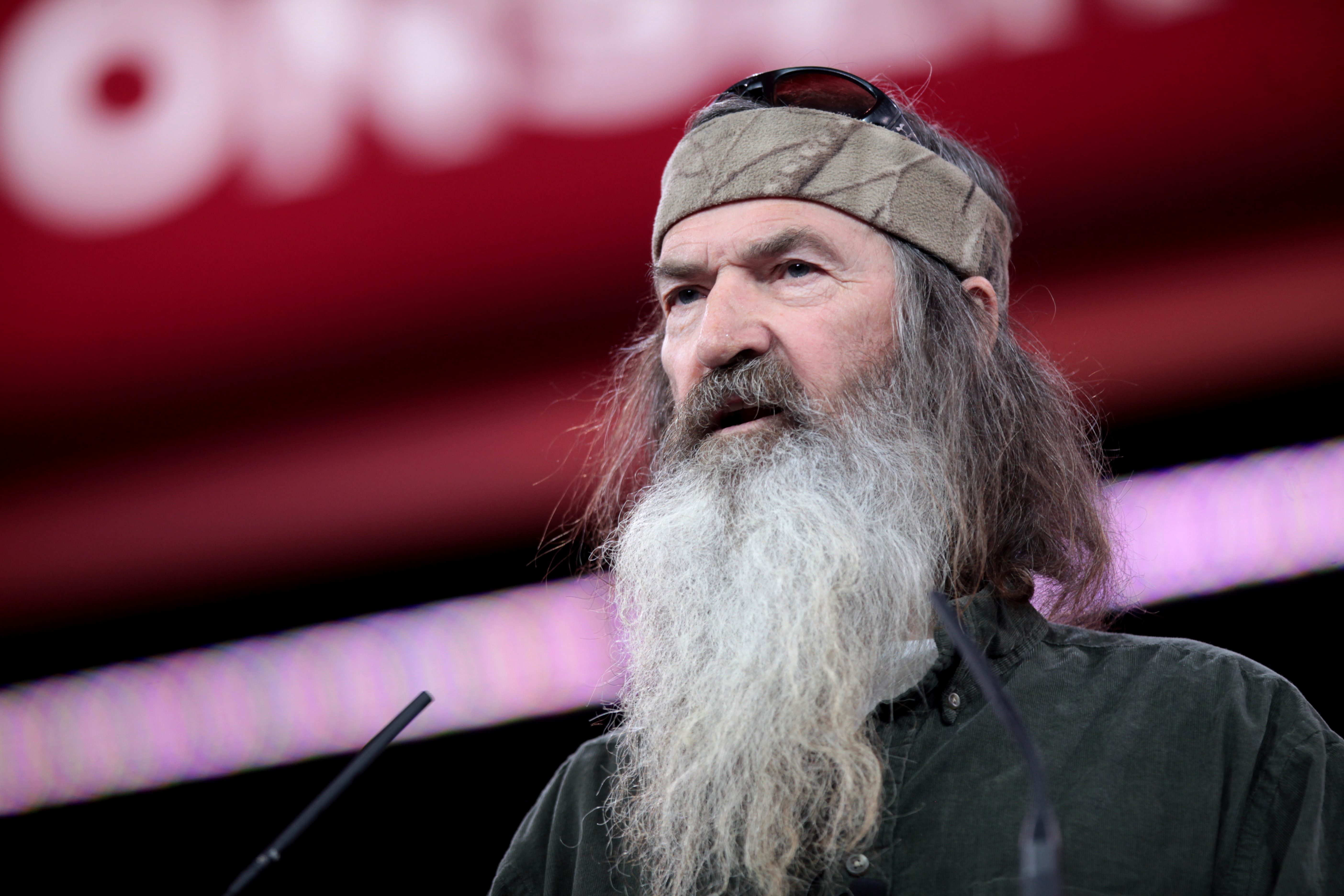The photograph is an up-close and clear capture of Phil Robertson, known from "Duck Dynasty." He appears to be speaking, as his mouth is open in mid-speech. Phil, who looks to be in his 70s, has a very long white scraggly beard that stretches down to his chest and a full mustache with streaks of gray. His hair is a mix of gray and dark, shoulder-length and unkempt. He wears an army green, possibly beige, hunting-type headband, about an inch thick, and black-framed sunglasses rest on top of his head. Phil is dressed in a faded black shirt or jacket, though the photo cuts off at his shoulders, making it unclear if the shirt has long or short sleeves. In front of him are two thin black microphones, appearing almost like straws. The background is blurred, but it features a sign with red, white, and black colors.